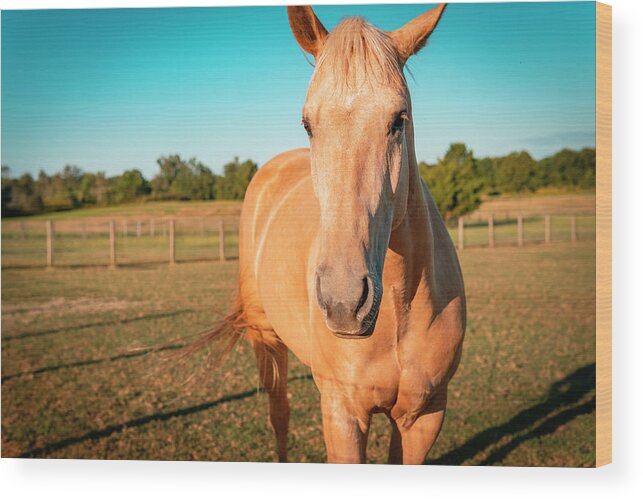This image, reminiscent of a photograph or perhaps a canvas, features a striking light brown horse standing head-on, facing the camera. The horse's ears are perked up attentively, and a portion of its tail is visible, swishing off to the side. To the right side of the image, there is a horizontal edge with a tan border and a white lining beneath it, creating depth and framing the scene.

The horse casts a distinct shadow of its legs towards the bottom right corner, while additional shadows are scattered across the grassy pasture it stands upon. Behind the horse, a fence with posts spaced about three to four feet apart stretches across the background, separating the pasture from a dense tree line. Above the trees, an open sky completes the serene landscape.